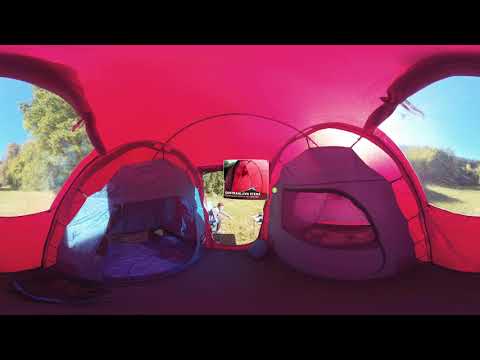The image captures the interior of a spacious, family-sized tent, predominantly colored in vibrant shades of red, yellow, and purple. The tent features a central entrance flanked by two zippered pod areas—small, semi-private sleeping nooks with purple-colored entrances and light purple floors. Additionally, two large plastic windows on either side of the entrance bathe the interior in sunlight. The backdrop visible through the open tent reveals lush greenery with trees and grass, indicating a serene, nature-filled setting. A small, superimposed picture with some unreadable writing is positioned between the vestibule doors, hinting that this image might be from a promotional material. The tent appears comfortable, accommodating three to four people, making it ideal for family camping trips.